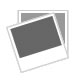This is a highly detailed, full-color image of a vertically rectangular book positioned on a light gray surface, taken indoors with artificial lighting that gleams on its shiny protective cover. The book's cover features a black background with prominent text and imagery. Dominating the top of the cover, in large, bold, uppercase orange letters, is the title, "HALLOWEEN 25." Superimposed across the number "25" in smaller, uppercase white text is the subtitle, "YEARS OF TERROR." Below the main image, in much smaller but still uppercase orange text matching the title, is the phrase, "A REVEALING LOOK AT THE CLASSIC HORROR SERIES." The central image on the cover is a stark black-and-white depiction of the infamous Michael Myers Halloween mask, characterized by hollow, dark eyes and a featureless, eerie face.